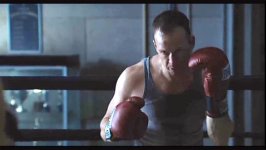This photograph depicts a white boxer practicing alone in a boxing ring, indicated by the shadow of ropes in the background. He appears to be in his 30s or 40s, with short black hair that is slightly receded in the front. The boxer is dressed in a blue or possibly gray tank top, and he is wearing red and black Everlast boxing gloves. He looks very sweaty, suggesting an intense workout session.

The small, rectangular image, approximately two by two or two by one and a half inches, does not contain any identifiers such as names or dates. The setting seems to be a dimly lit gym, as indicated by the lighting conditions described. Behind the boxer is a trophy case with a glass front and white sides, containing gold cup-shaped trophies and some with wooden bases, though the details are somewhat blurred and difficult to read. Above the trophy case, there's a blue poster, potentially listing the names of the trophy winners. The background features light stone paneling, adding to the gym-like atmosphere of the scene.